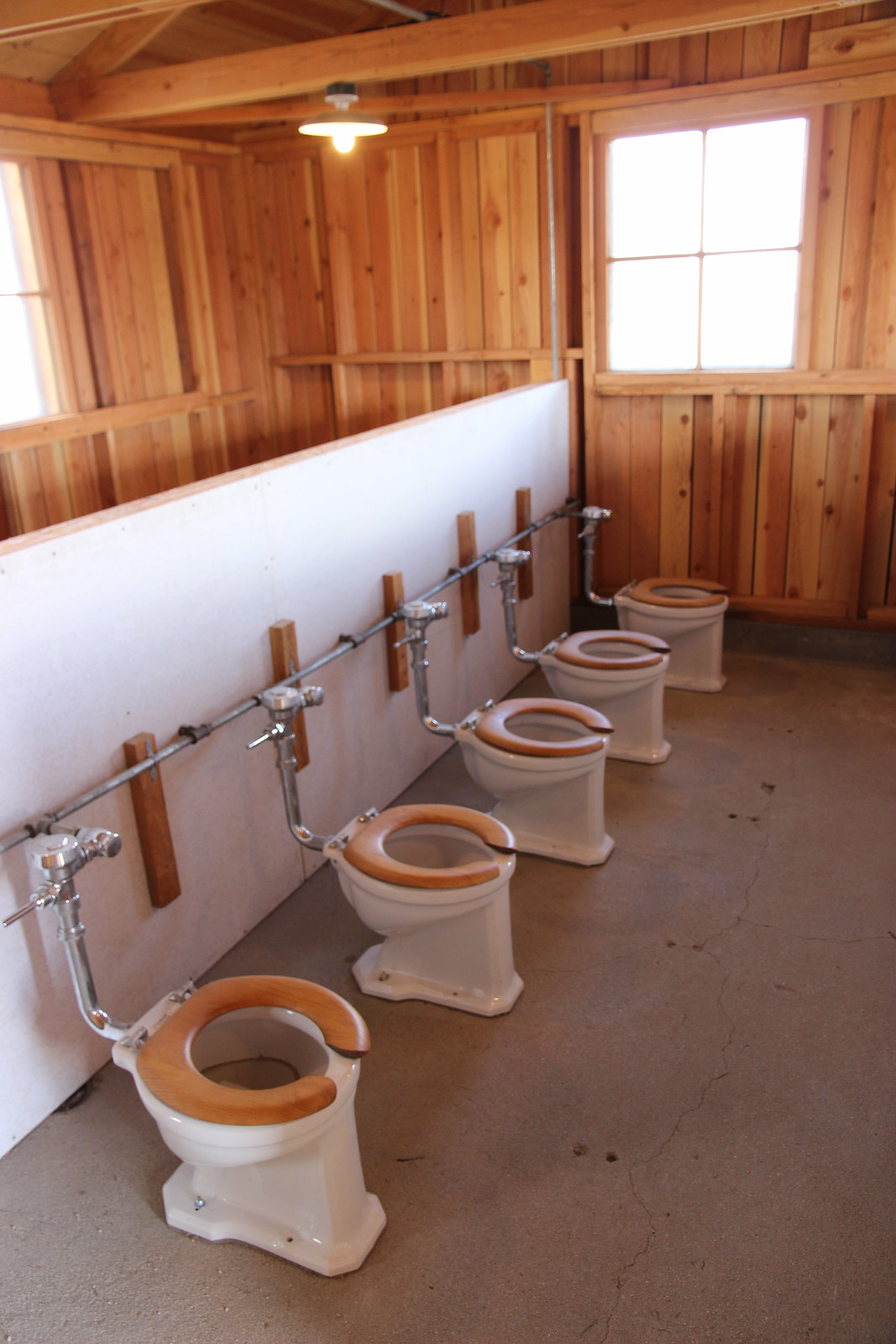This image depicts a perplexing public restroom setup, with five white toilets lined up side by side, each featuring a brown wooden seat. The lack of dividers or walls between the toilets means there's no privacy, a key factor typically desired in such settings. The toilets are attached to a white half wall, which has a single pipe running across it, connecting all the fixtures. The room's interior appears to be newly constructed, with brown wood paneling reminiscent of cedar and wooden beams on the ceiling. The space includes a couple of windows and a light fixture on the ceiling, and the floor is made of concrete. The environment is reminiscent of a wendy house but unexpectedly functions as an open-concept restroom.